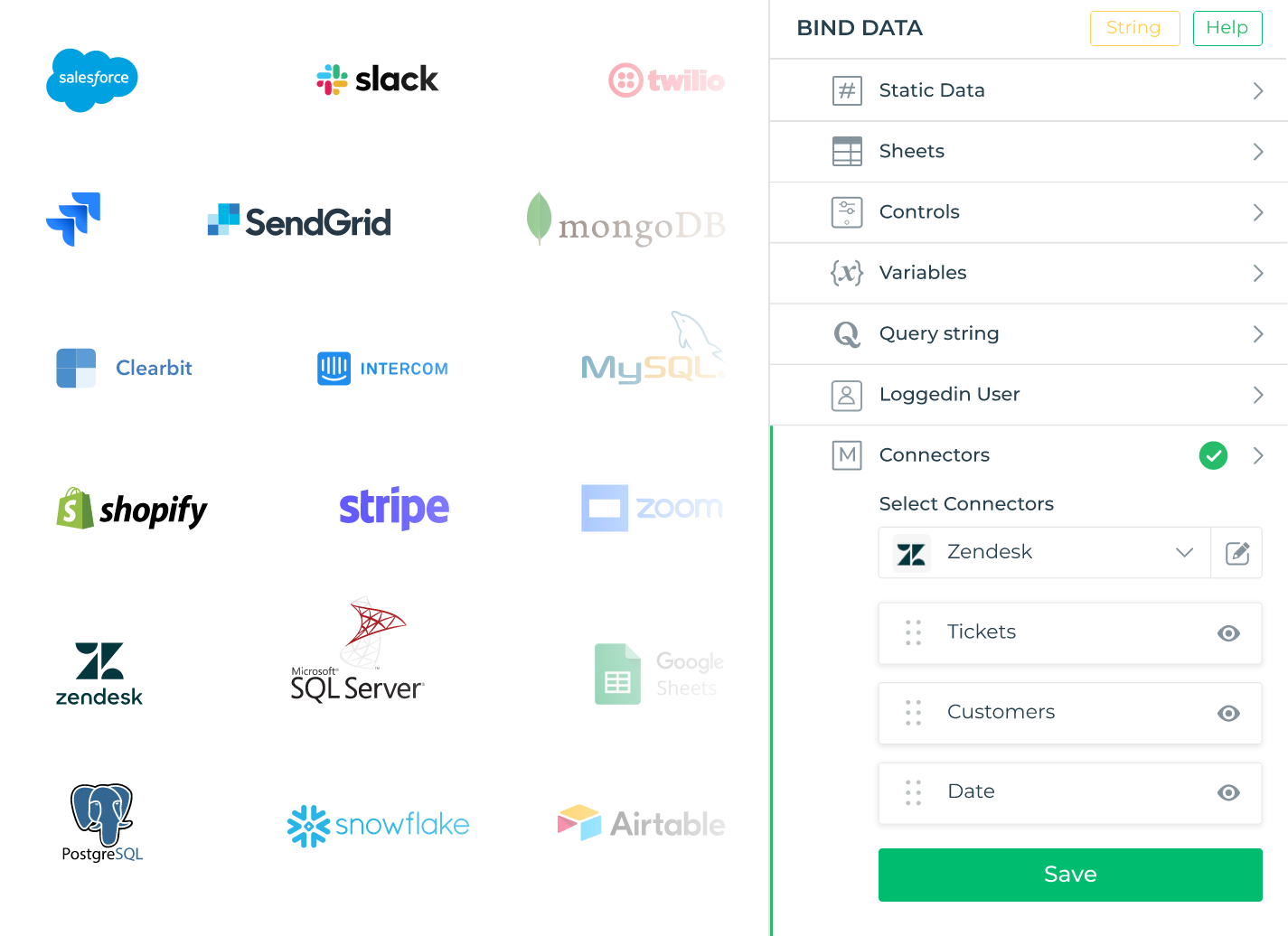The image showcases a user interface with a variety of icons aligned on the left side, though they are somewhat blurry and difficult to identify at a glance. The legible icons among them are Slack, Twilio, SendGrid, MongoDB, Clearbit, Intercom, MySQL, Shopify, Stripe, Zoom, Zendesk, SQL Server, Snowflake, and Airtable. 

On the right side of the interface, there is a section titled "Bind Data." Within this section, there is an orange button labeled "Bind Data" and a green button labeled "Help." Below these buttons, several options are listed: "Static Data," "Sheets," "Controls," "Variables," "Query String," "Logged-in User," and "Connectors."

Next to "Connectors," there is a green circle with a checkmark inside it, indicating that connectors are active or verified. Beneath this, the text "Select Connectors" appears, followed by a box containing the word "Zendesk" with options such as "Tickets," "Customers," and "Date" listed underneath it.